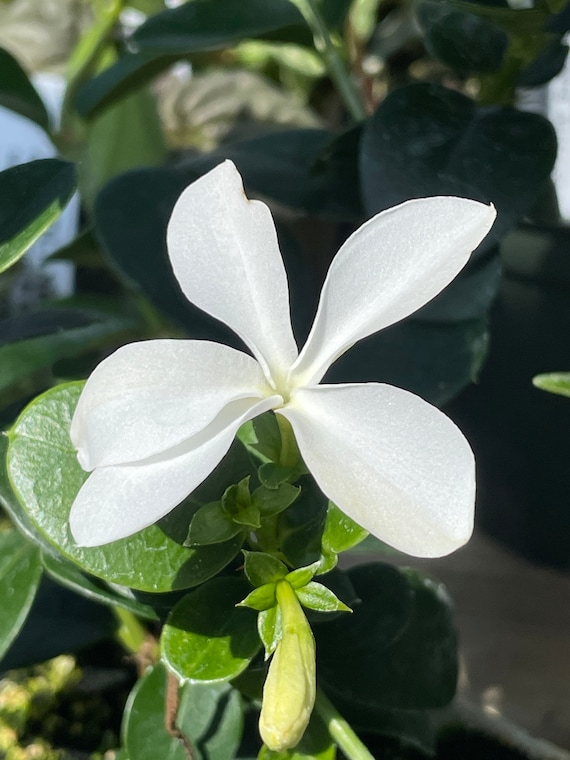The photograph captures a close-up of a single, stunning white flower partially in bloom, featuring five long, oblong silky petals that radiate gracefully towards the viewer. This delicate flower, resembling a lotus, stands prominently on a stem adorned with small green leaves. In the foreground, a not-yet-opened flower bud points southwards, hinting at the plant's continuing cycle of blooming. The flower and the leaves on the stem are bathed in direct sunlight, which accentuates the fine textures of the petals and leaves. The shaded background, featuring large, blurry leaves, contrasts against the crisp clarity of the main flower, adding depth to the image. In the top left corner, hints of another potential lotus flower peek through, enriching the scene with botanical layers.